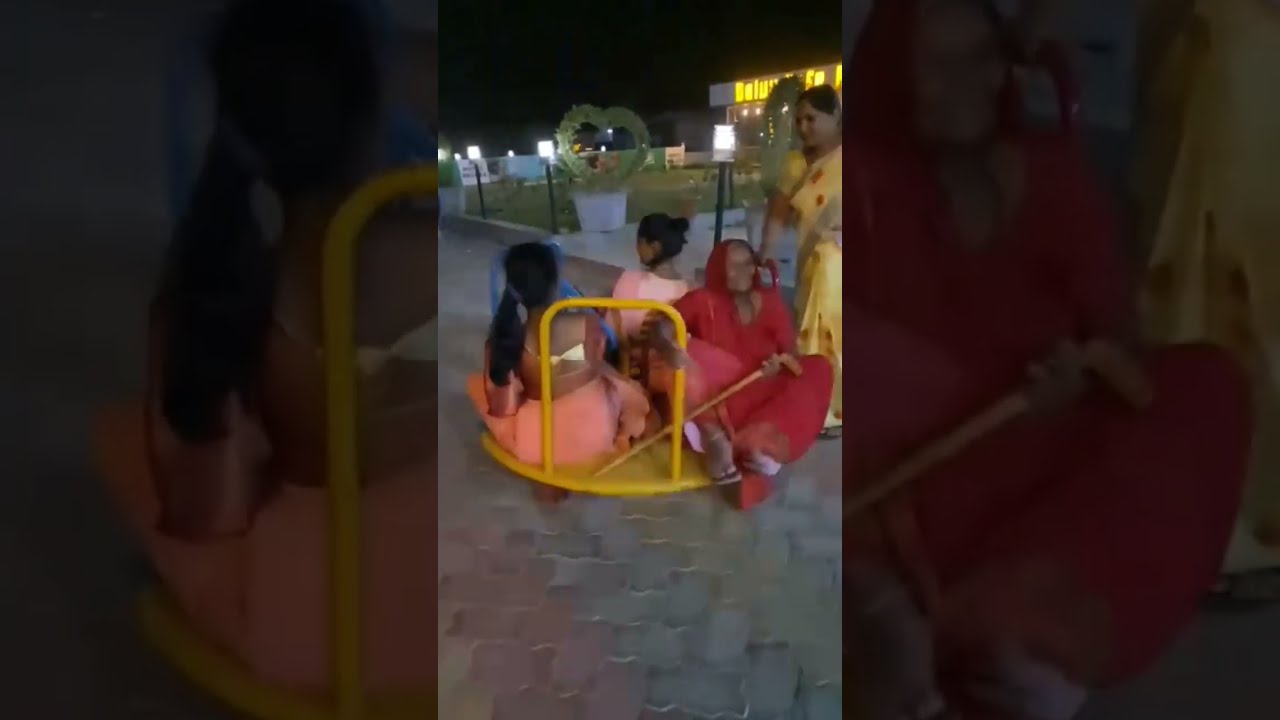This is a complex image featuring a horizontal rectangular photograph with the central part showing clear details, flanked by two dark, partially transparent bands on either side. The photograph depicts a nighttime outdoor scene on a brick-paved street, enhanced by several lights lining the pathway. At the center of the image, three people are seated on a circular yellow cart with a large handle. The individual in the middle, dressed entirely in red with a hood, appears to be an older woman, possibly homeless, using a brown cane for support and surrounded by her belongings, including an orange container in front of a small dog. Flanking the seated individuals to the right stands a young woman in a yellow dress, holding onto the cart. The scene is set against the backdrop of a two-story building, and features a heart-shaped flower pot sculpture. The image includes additional details such as a yellow neon sign in the upper right corner and a room or area filled with packages in the background, suggesting a possible warehouse setting.